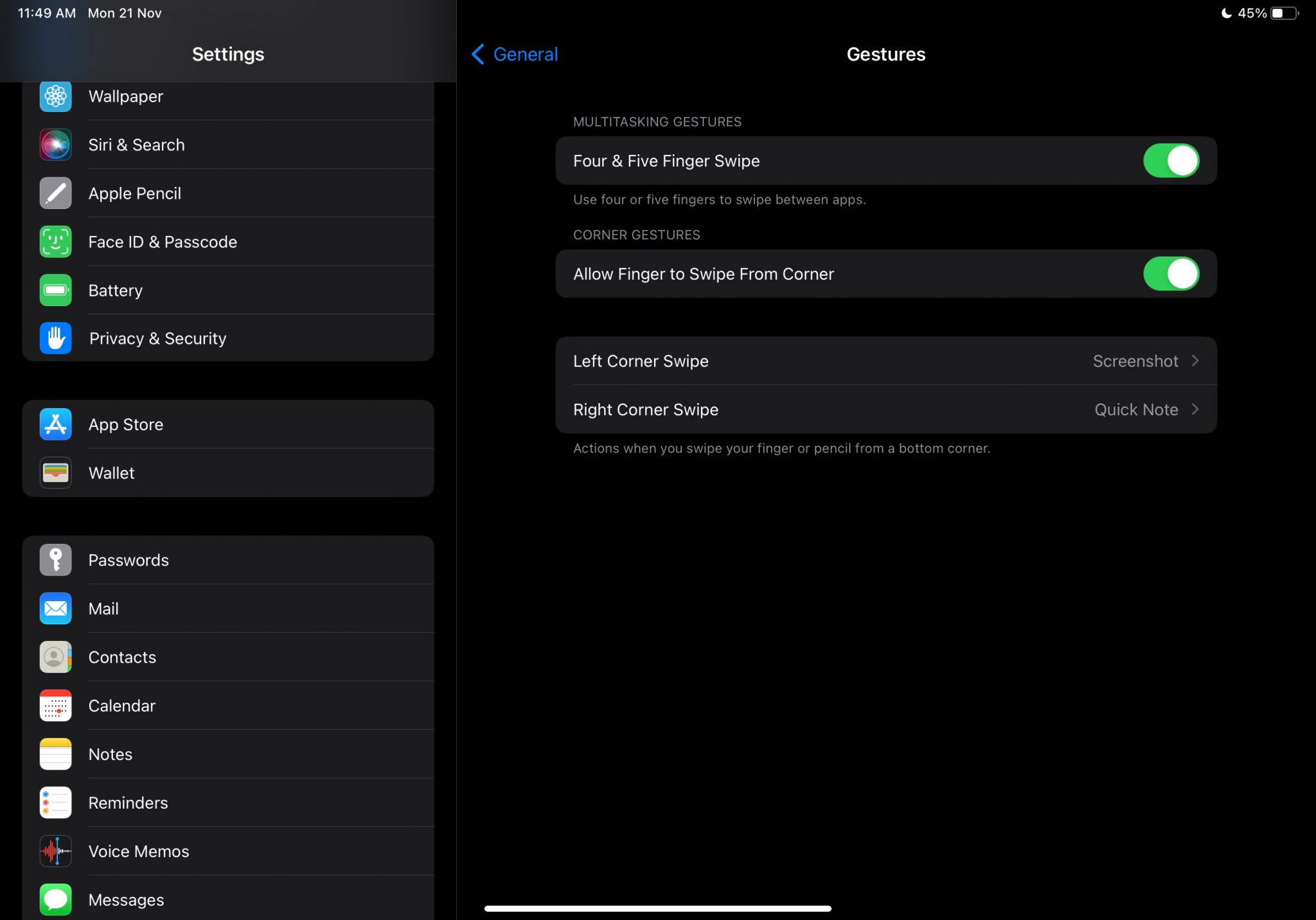A screenshot of a dark-themed settings menu from a mobile device. The image displays a black background with white text and colorful icons.

At the top of the screen:
- Battery life: "45%" (white text)
- "Do Not Disturb" mode icon
- Timestamp: "11:49 a.m."
- Day and date: "Monday, November 21st"

Directly beneath the top bar, the word "Settings" is prominently displayed in white.

The settings menu includes the following options, each accompanied by distinct icons on the left side, varying in blue, green, gray, multicolors, and some white with red or yellow:
- Wallpaper
- Siri & Search (multicolored icon)
- Apple Pencil
- Face ID & Passcode
- Battery
- Privacy & Security
- App Store
- Wallet
- Passwords
- Mail
- Contacts
- Calendar
- Notes
- Reminders
- Voice Memos
- Messages

On the right side of the screen, a section labeled "Gestures" is visible.
- The word "General" appears in blue with an arrow pointing left.

Under "Gestures," the following options are listed:
- "Multitasking Gestures"
  - "Four or Five Fingers Swipe": Allows using four or five fingers to swipe between apps (The text about "APAS" is unclear).
  - Both this option and "Corner Gestures" are highlighted with a green switch indicating they are turned on.
- "Corner Gestures": Allows swiping from the corner (also switched on in green).

Details under "Corner Gestures":
- "Left Corner Swipe"
  - Right option: "Screenshot"
- "Right Corner Swipe"
  - Right option: "Quick Note"
  - Small text description: "Actions when you swipe your finger or pencil from a bottom corner."

The overall interface is clean and organized, with functional features prominently displayed for easy navigation.